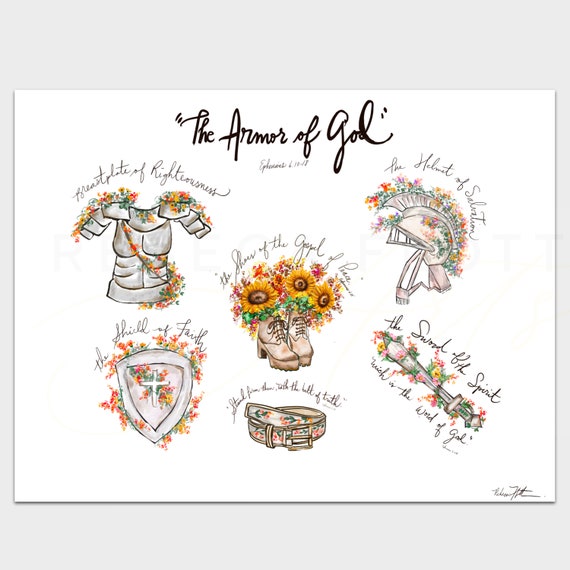On a light blue-gray background, a visually stunning digital graphic titled "The Armor of God" is presented in elegant cursive font at the top, with an unreadable line below. The image is framed with a decorative border and centers around a white rectangle that neatly organizes the different elements of the armor, each infused with intricate, feminine floral designs. 

On the left, below the title, a silvery-gray chest shield adorned with flowers is labeled, “Breastplate of Righteousness.” Directly below, a shield featuring a cross and floral embellishments is identified as, “The Shield of Faith.” Moving to the center, a pair of almost granny-style boots, with vibrant sunflowers and other colorful flowers sprouting from them, represent “The Shoes of the Gospel of Peace.”

To the right, “The Helmet of Salvation” showcases a helmet gracefully decorated with flowers. Below the helmet, an intricately designed belt with ivory, green, and pink floral patterns appears, though the label is too small to read clearly. The final element, “The Sword of the Spirit, which is the Word of God,” depicts a sword exquisitely wrapped in a variety of flowers, emphasizing the beauty and power of faith.

Collectively, this piece transforms traditional armor into a symbol of faith and spirituality, merging historical elements with artistic and religious significance.